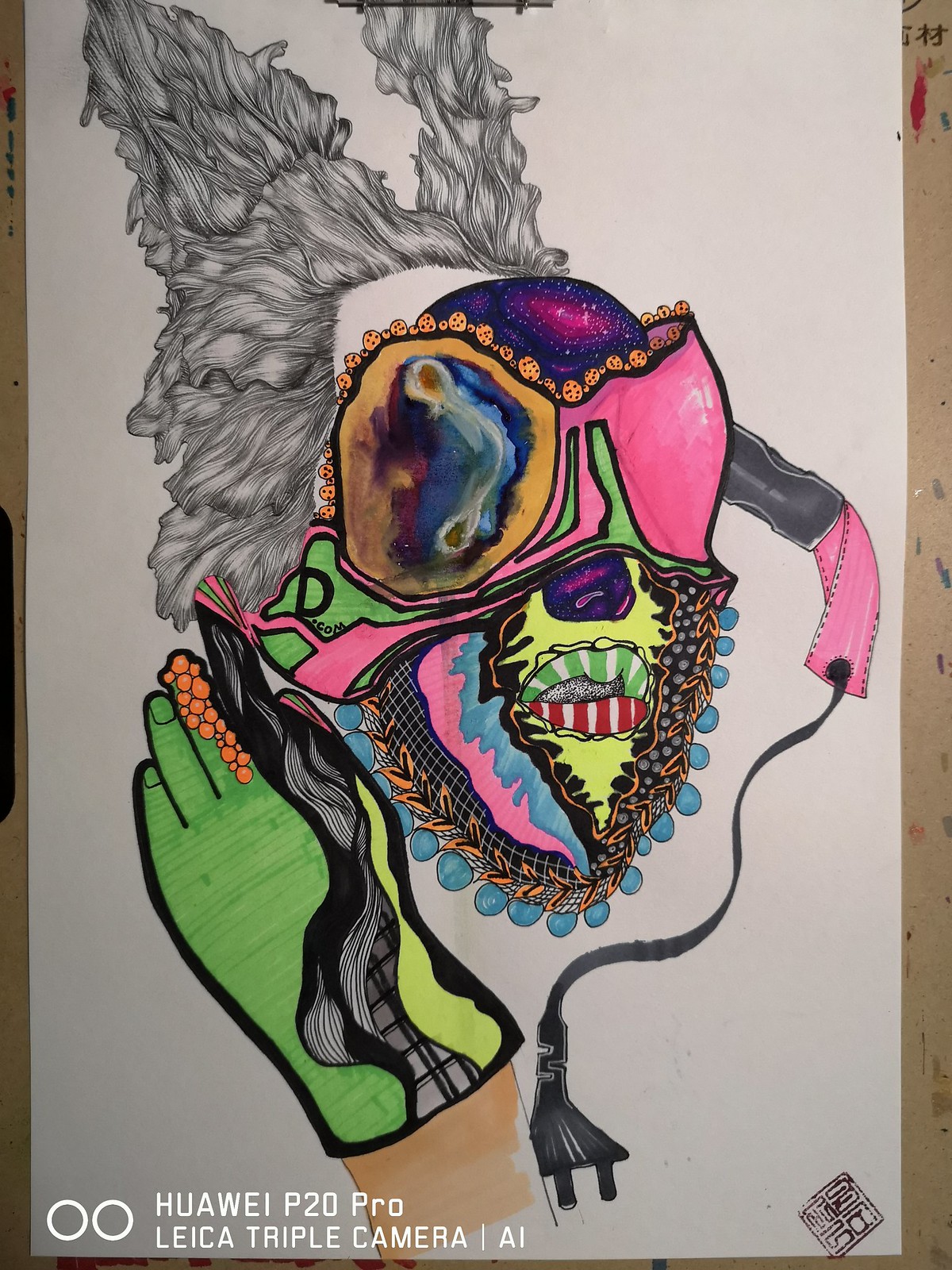The image is a vibrant and intricate piece of multimedia artwork featuring a blend of various artistic techniques and materials. The central focus appears to be a human face adorned with what looks like goggles or a mask. The medium utilized includes ink, pen, acrylic marker, and possibly alcohol ink, creating a swirling, dynamic effect throughout the piece.

The composition is rich in texture and color, showcasing a plethora of shades such as orange, pink, yellow, green, and blue. Different textures can be identified within the artwork, including patterns reminiscent of a galaxy, nebula, grid formations, and delicate, leaf-like structures that seem to form both the hair and hand of the figure. The hand, in particular, appears less refined compared to the rest of the piece, with an anatomically incorrect and somewhat childlike depiction that contrasts starkly against the more sophisticated elements.

The artwork is presented on a simple white piece of paper, akin to standard printer paper, which underscores the raw and unpretentious nature of the piece. In the bottom right corner, there is a distinct seal or stamp alongside a logo that reads "Huawei P20 Pro Leica Triple Camera AI." This suggests that the image may have been captured or edited using this specific camera technology.